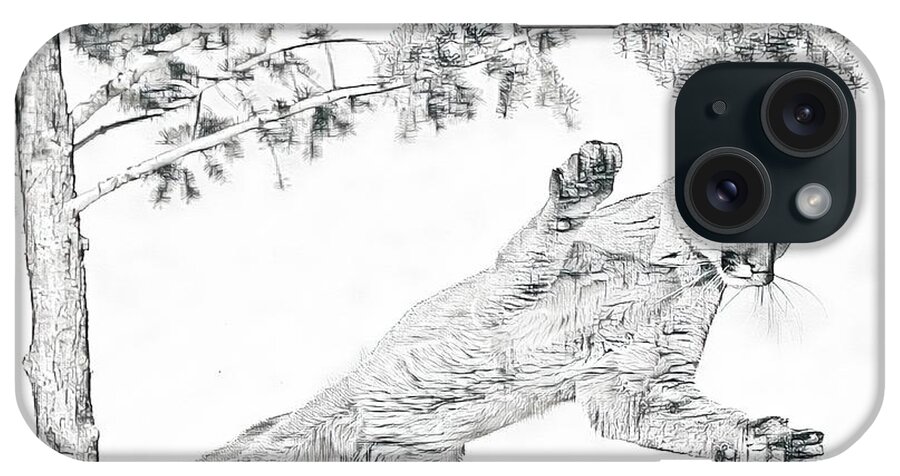The image portrays the back of an Apple iPhone placed on its side, longer from left to right. The iPhone case features a black and white illustration, predominantly white, with the artistic depiction of a cougar or mountain lion. The animal's head is cut off by the phone's two large camera lenses located in the upper right corner, revealing only its snout, whiskers, and outstretched paws as if it's leaping downward. To the left of the leaping cougar is the detailed trunk and branches of an evergreen tree, completing the monochromatic design. The camera setup also includes a smaller lens-like element, and there's another small, round component in the upper left corner.